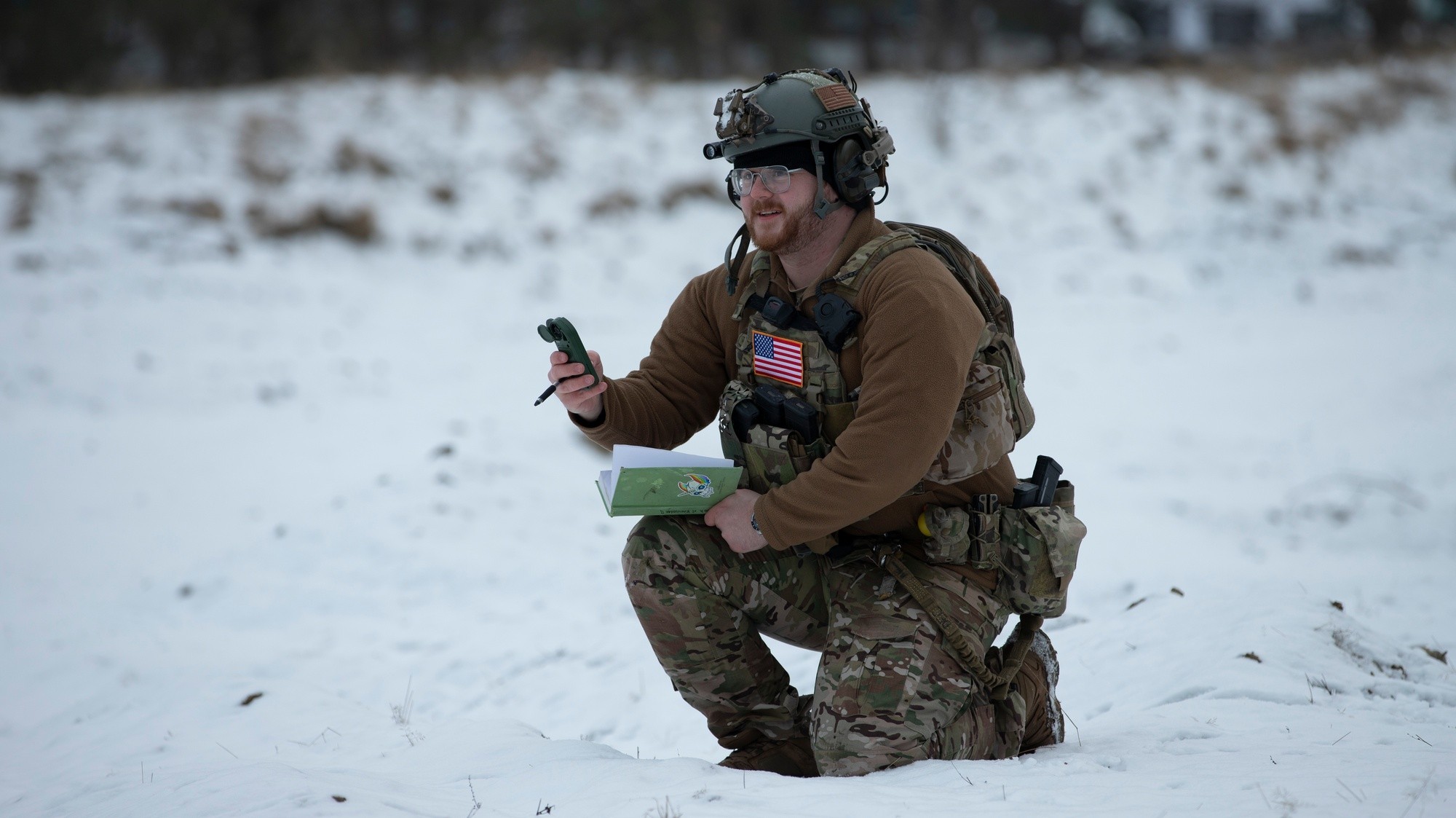In the center of a snow-covered forest, an American soldier is depicted in sharp focus, crouching with his left knee on the ground and his right knee bent behind him. The background is blurred, featuring a tree line and a small hill with patches of grass poking through the snow. Scattered rocks dot the snowy field around him. The soldier wears a green helmet with a black beanie underneath and glasses that frame his orange-yellow beard and mustache. His military attire includes a camouflage chest plate over a brown long-sleeve shirt, camouflage pants, and a belt with several utility pouches on his left hip. An American flag is prominently displayed on his chest. He holds an open green book with his left hand, adorned with a small cartoon character sticker, while his right hand holds a device that appears to be for navigation or detection. The soldier is slightly smiling, appearing focused yet calm as he looks forward.